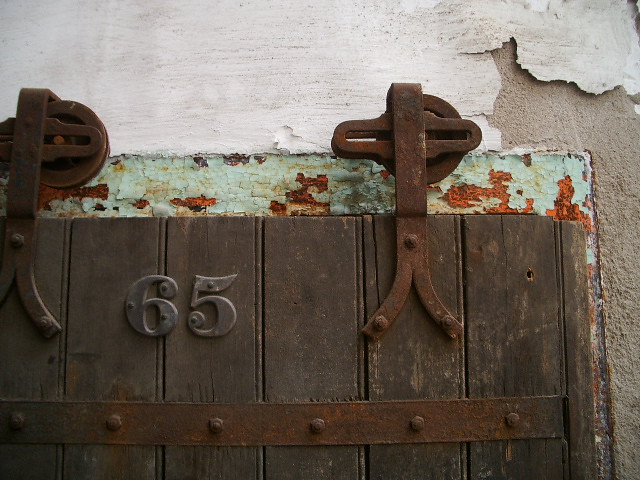This outdoor image captures a rustic wooden door embedded within a concrete wall that's partially coated with peeling stucco paint. Starting from the upper left-hand side, the stucco appears white but is visibly flaking, revealing the bare concrete underneath. The door is framed by a rusting metal structure, suggesting prolonged exposure to the elements. Attached to this frame are two rusty metal straps, each featuring wheels at the top, likely serving to stabilize the door and prevent it from slamming. These straps, heavily oxidized, are anchored with lug nuts.

The wooden door itself, which has a vertical slat design and a deep brown hue, is central to the image. Prominently displayed in the middle of the door are the metal numerals "65," affixed with visible screws. A rusted metal band runs horizontally across the bottom part of the door, dotted with rivets or screws. The overall weathered appearance of both the door and its frame, coupled with the deteriorating wall paint, gives the image a distinctly aged and rugged character.